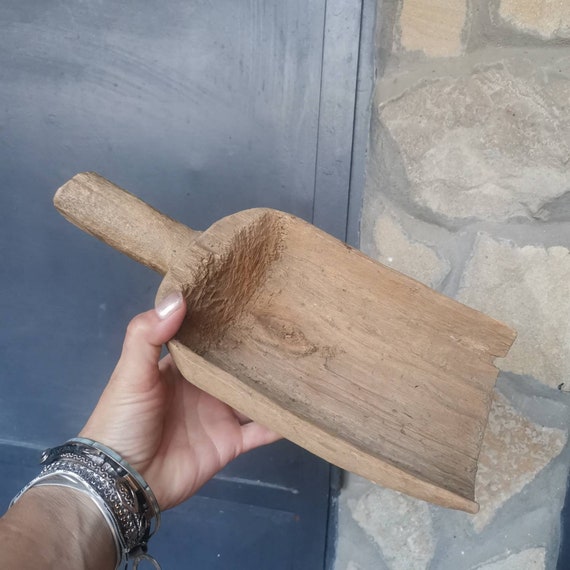An up-close square-shaped photograph captures a left hand with an abundance of silver bracelets, belonging to a person who appears to be of lighter skin, holding what resembles an old, handmade, wooden dustpan or scoop. The item is made from one solid piece of wood, with a short handle and an angled scoop. The background features a black or dark gray door on the left and a gray, stuccoed wall composed of large light gray stones on the right. The setting seems to be the exterior of a home or building.